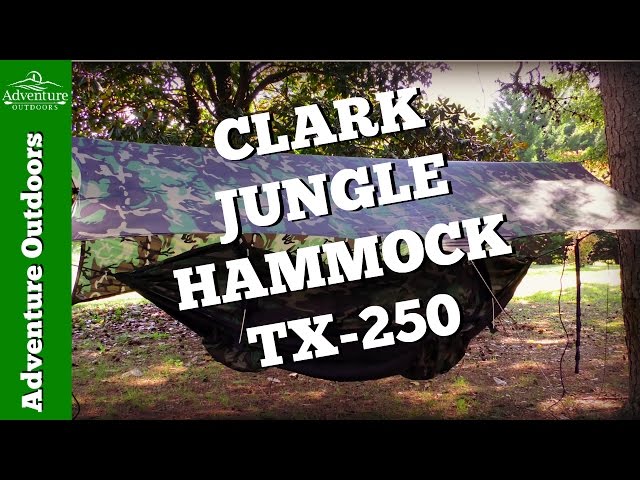This image resembles a YouTube thumbnail and serves as an advertisement for the Clark Jungle Hammock TX-250. On the far left side, there's a rectangular green banner with a white mountain logo at the top, featuring the text "Adventure Outdoors" both horizontally at the top and vertically along the banner. The main scene appears to be shot in a backyard, displaying elements such as trees and green leaves in the background, patches of dirt and grass on the ground, and a wooden log on the right. Central to the image is a dark-colored hammock with a camouflage sunscreen above it, suspended between two poles. Diagonally across the middle of the image, the product name "Clark Jungle Hammock TX-250" is prominently displayed in white text.